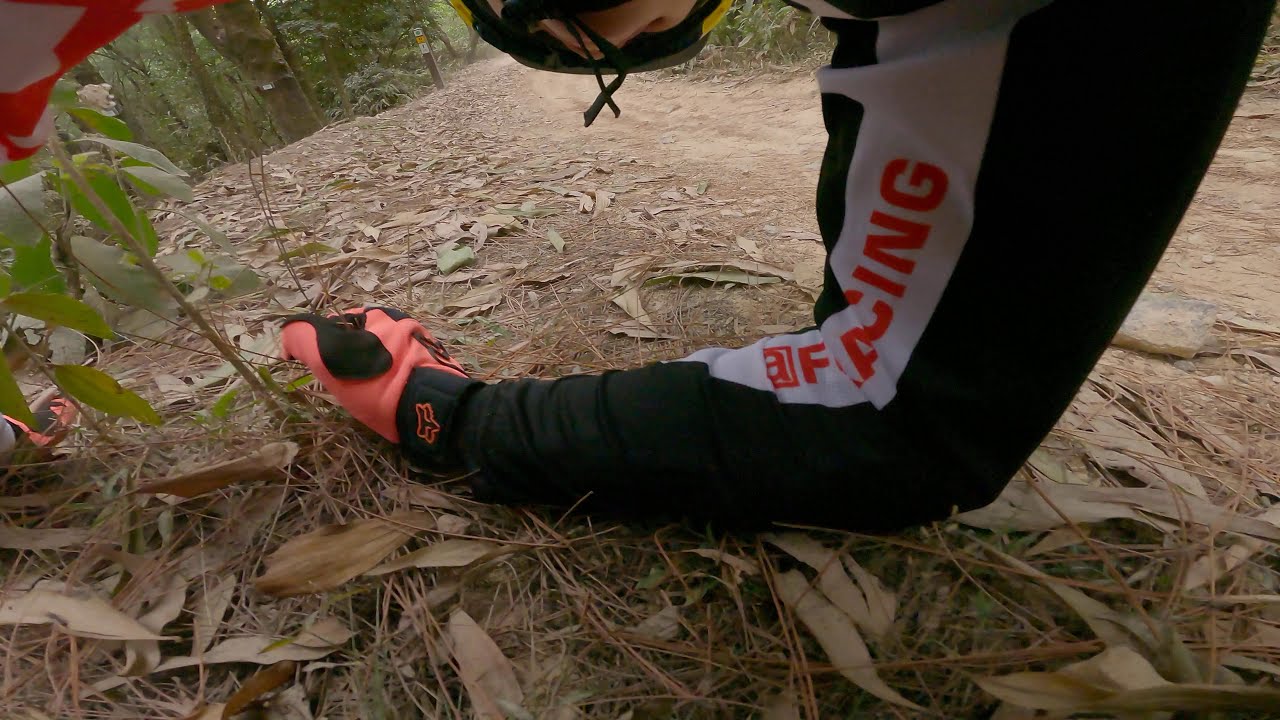The image depicts a person, likely involved in motorsports, leaning down on a trail covered with dead pine needles and leaves. The individual's left arm, clad in a black long sleeve with a white stripe and partially readable orange lettering possibly spelling out "racing" or "off-roading," is bent and supporting their body on the ground. The orange glove on this hand features a recognizable Fox Motorsports logo, and the glove's black cuff also has some unreadable orange text. The person's head is partially visible, adorned with a black helmet. In the background, there's a mix of light brown dirt and rock, alongside some sickly-looking trees with sparse green foliage. The rock, bearing a pointed shape, is surrounded by what appears to be green leaves or possibly water, capped with a red stripe. The scene suggests a moment of pause or rest, perhaps after a motorsport activity.